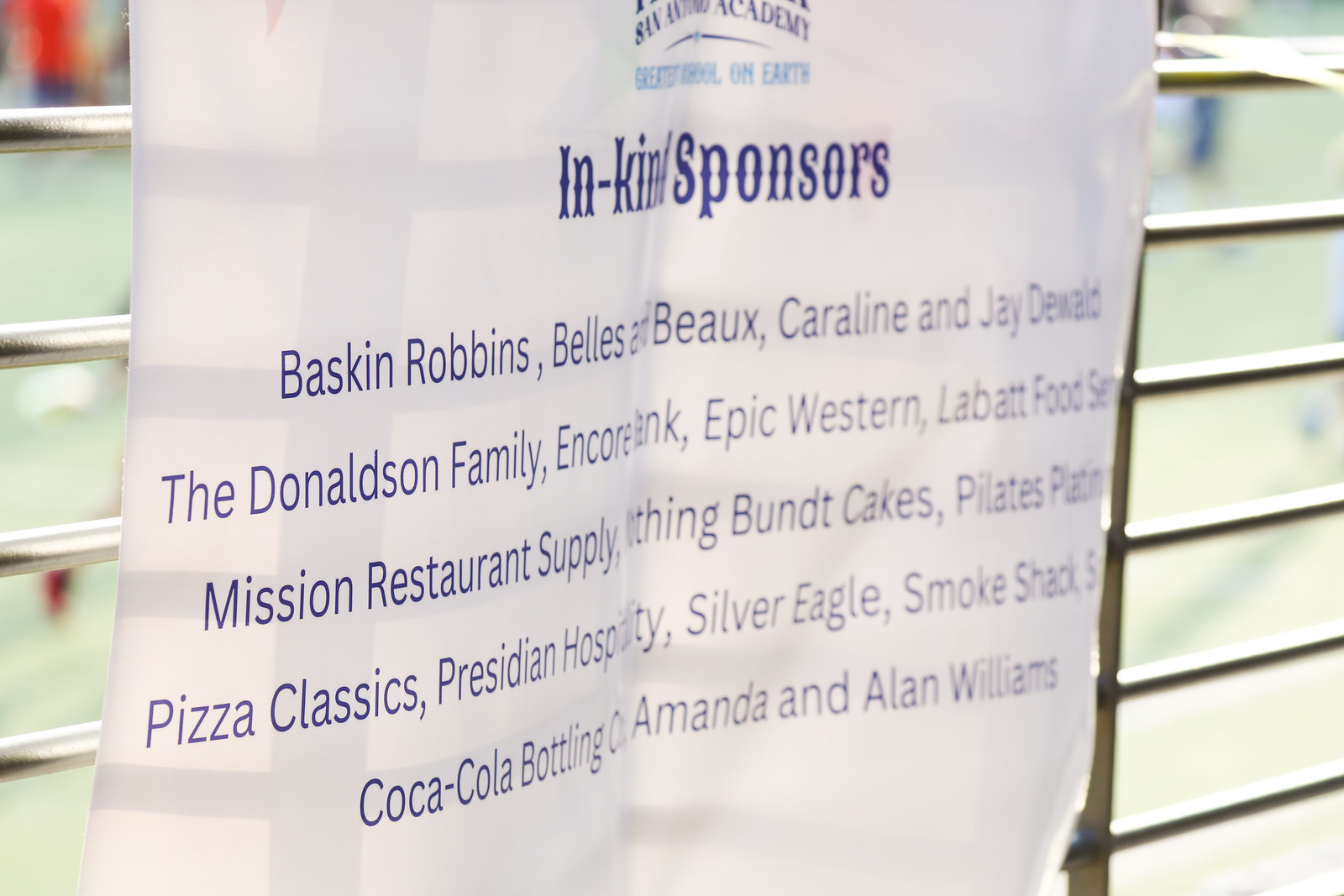This horizontally oriented photograph captures a white, somewhat transparent sign attached to a silver metal gate, consisting of evenly spaced horizontal metal poles. The sign prominently displays "In-Kind Sponsors" in large blue letters beneath a logo at the top. A list of sponsors follows, though some words are cut off or partially obscured, including names like "Baskin Robbins," "Bell & Bow," "Caroline and Jay DeWald," "The Donaldson Family," "Encore Bank," "Epic Western," "Labatt Food Service," "Mission Ready Supply," "Nothing Bundt Cakes," and "Pilates Plating." Additional sponsors mentioned are "Pizza Classics," "Poseidon Hospitality," "Silver Eagle," "Smoke Shack," and "Coca-Cola Bottling Co." The sign's surface shows shadows of the metal poles behind it, adding to the texture, while the photo's angled perspective and slight creasing of the sign make some text difficult to decipher. The backdrop appears outdoors, offering a blurred view of fencing to the right.